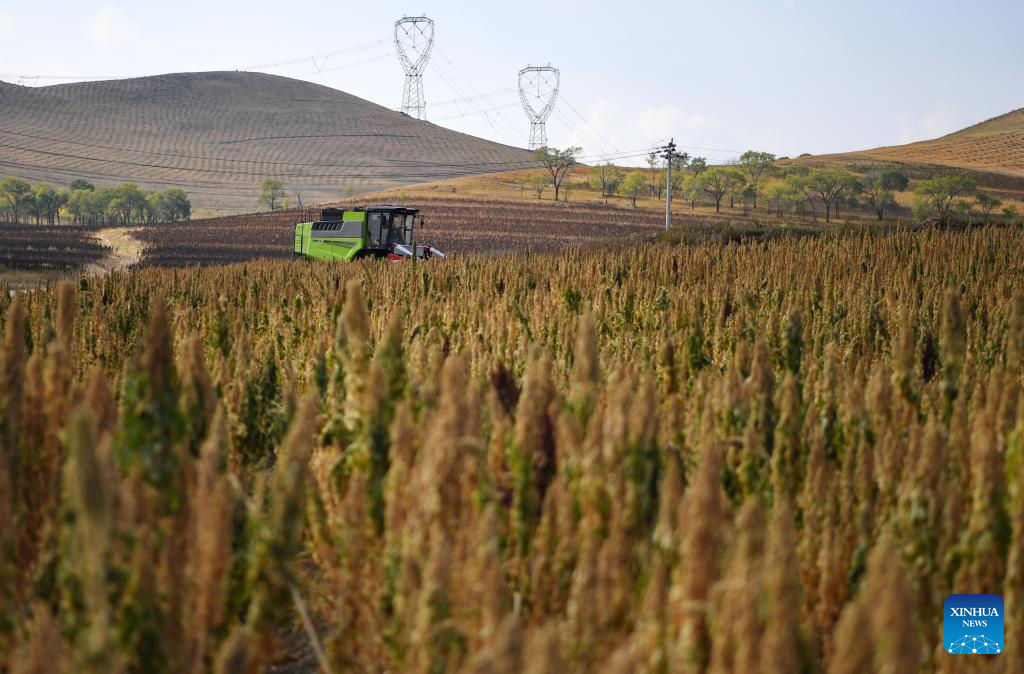The photograph captures a picturesque, panoramic view of a vast agricultural landscape, characterized by gently rolling hills sparsely adorned with small clusters of trees. Dominating the foreground are long, tapered plants that resemble wheat, their tips tinged reddish-brown and foliage vibrant green. The proximity of these plants causes a slight blurriness in the photo's foreground. A prominent feature in the midground is a large green tractor with red accents and a glass cab, actively working the fields. The horizon showcases a mix of natural and man-made elements, with a few scattered trees and two prominent power line towers alongside a solitary telephone line. The sky above is a bright, light blue, adding to the serene ambiance of the scene. In the bottom right corner, a blue logo reads "Xinhua News," indicating the image's origin from a Chinese news source.